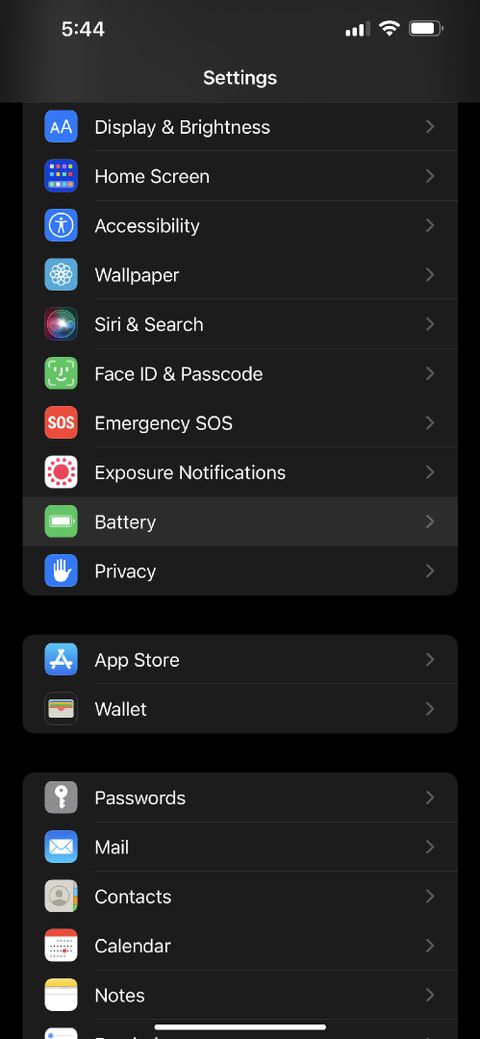This image is a screenshot taken from the settings page of an iPhone operating in dark mode, where the background is entirely black. At the very top left corner, the time is displayed in white, reading '5:44'. In the top right corner, the status indicators show three out of four bars of cellular connectivity, full Wi-Fi signal, and a battery level at 56%.

In the center of the top section, the title 'Settings' is prominently displayed in white text. The first visible section of the settings menu starts with 'Display & Brightness', followed by options for 'Home Screen', 'Accessibility', 'Wallpaper', 'Siri & Search', 'Face ID & Passcode', 'Emergency SOS', 'Exposure Notifications', 'Battery', and 'Privacy'. Each of these options is accompanied by a corresponding icon to the left and a right-pointing arrow to the right, all set against the dark background with their labels in white text.

- 'Display & Brightness' is represented by an icon featuring two letter 'A's of differing sizes on a blue background.
- 'Wallpaper' displays a white flower on a light blue background.
- 'Emergency SOS' is marked with a red background and the letters 'SOS' in white.

Following this main block of settings options, there's a second block featuring 'App Store' and 'Wallet', again with respective icons and right-pointing arrows. Below this is a third block that shows icons and labels for 'Passwords', 'Mail', 'Contacts', 'Calendar', and 'Notes', although the view of this section is cut off at the bottom of the screenshot.

At the very bottom of the screen, a thin white bar is visible, indicating that a swipe up gesture will return the user to the Home Screen. Overall, the black background makes the white text and colorful icons appear vivid and easily readable.